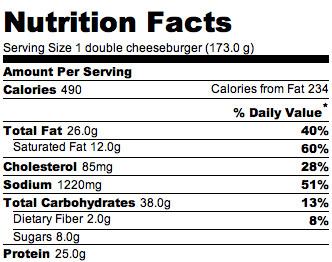This image depicts a Nutrition Facts label on a white background. At the top, it displays "Nutrition Facts" in bold black text. Directly underneath, smaller black letters state "Serving size: one double cheeseburger (173.0 grams)." A thick black line separates this from the next section, which reads "Amount per serving" in bold lettering. Below this, the label lists "Calories: 490" and "Calories from fat: 234."

Further details on the left-hand side include the following nutritional information, accompanied by their respective percentage daily values on the right:
- Total fat: 26.0 grams (40%)
- Saturated fat: 12.0 grams (60%)
- Cholesterol: 85 milligrams (28%)
- Sodium: 1220 milligrams (51%)
- Total carbohydrates: 38.0 grams (13%)
- Dietary fiber: 2.0 grams (8%)
- Sugars: 8.0 grams
- Protein: 25.0 grams

The entire label is presented in a clean, black and white format, maintaining a straightforward and easy-to-read layout against the white background.